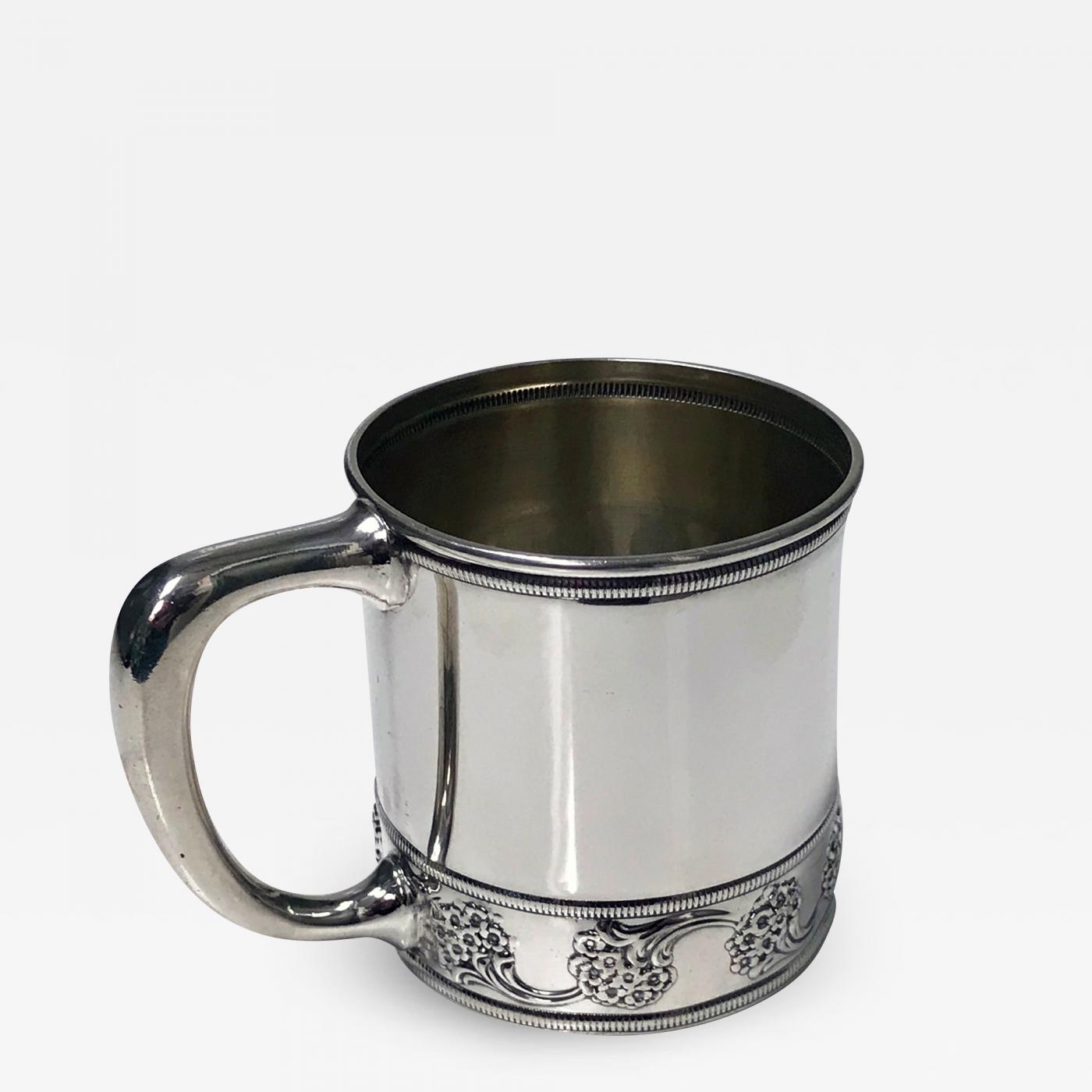This photograph captures a close-up of a silver metal mug set against a stark white background, giving it a product image feel. The entire mug, including the interior, is made of polished silver metal. The handle is large and smooth, resembling a coffee cup handle, with a C-shaped curve that reflects the surroundings. The mug features intricate decorative details that enhance its vintage, possibly Victorian style. 

Starting at the top rim, there is an embossed chain-like pattern with small circular rivets encircling the mug, adding a textured border. The bottom quarter of the mug displays a detailed, repeating floral design that includes small bouquets with stems and petaled flowers, each flower having a small black center. This floral pattern appears to swirl and intertwine around the base of the mug, bordered by similar chain-like ridges both at the top and bottom of the floral section. The interior of the mug showcases a brushed aluminum look, darker than the shiny exterior. The mug is clean and reflective, with its metallic texture capturing the light and creating subtle reflections of its surroundings. Through the opening at the top, the smooth, unadorned interior is visible, complementing the ornate exterior designs.